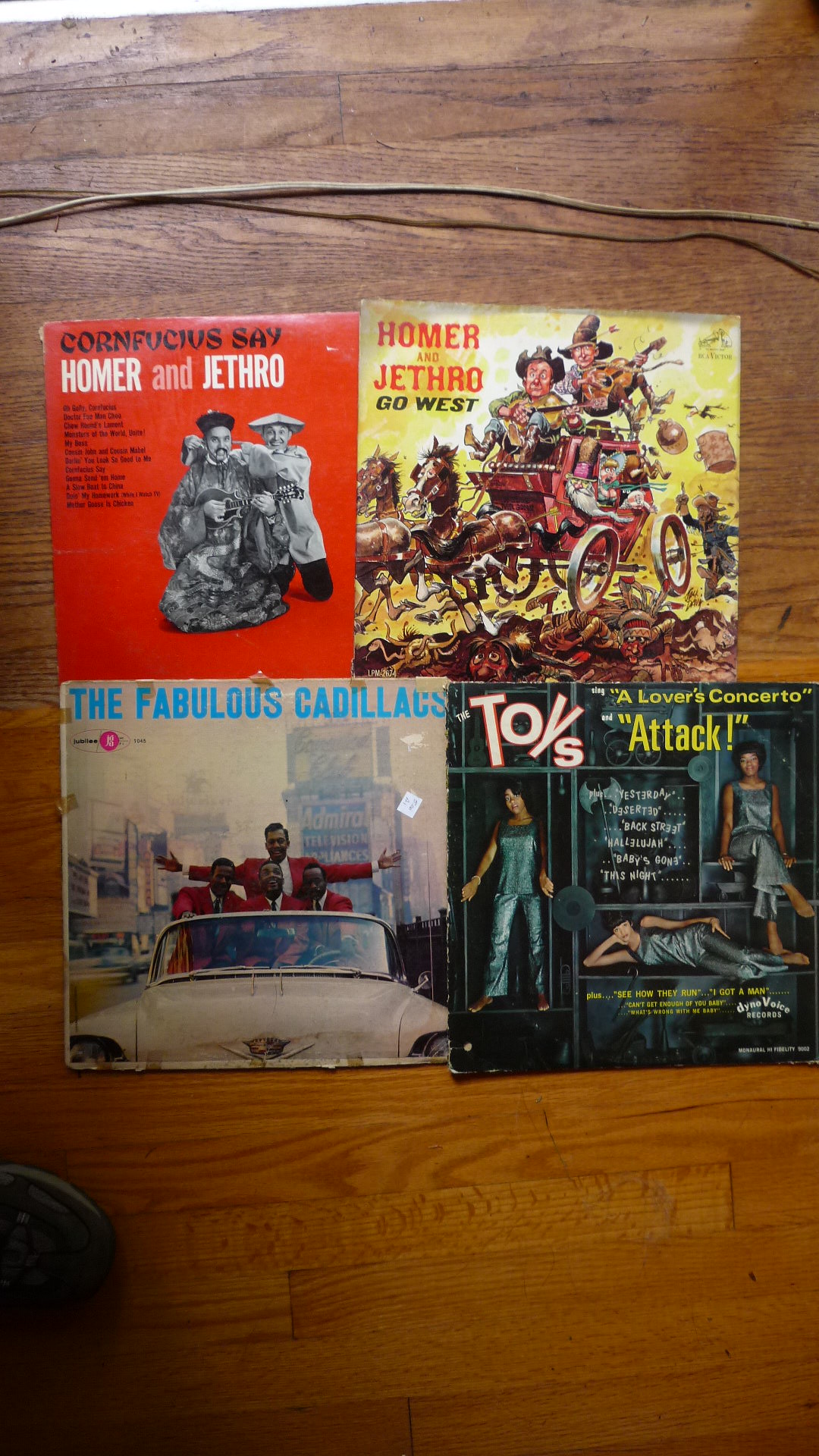This detailed photograph showcases four vintage record album covers meticulously arranged in a square formation on a medium-tone oak wooden floor. A horizontal cord casts a shadow over the image's upper section, suggesting a flash was used during capture. Intriguingly, the tip of the photographer's foot is faintly visible in the lower left corner.

The top-left album, titled "Confucius Say Homer and Jethro," features a vivid red background with a black-and-white illustration of two individuals in traditional Chinese attire. To its right, "Homer and Jethro Go West" displays a whimsical cartoon of an old-style wagon cart, complete with two guitar-playing figures and flying paraphernalia, pulled by two horses in a western setting.

Below, the bottom-left album, "The Fabulous Cadillacs," depicts a white convertible Cadillac with its windscreen visible. Surrounding the car are four black men in sharp red suits, standing in front of a misty cityscape with one man standing behind the front three, his arms outstretched.

The bottom-right album, titled "Toys, A Love Concerto, Attack!", boasts a dynamic layout with a glamorous woman in a shiny, silvery dress embroidered with "dino voice." The album cover lists several songs and features toy figurines that add a playful touch to the sophisticated design.

Each album cover is captured in exquisite detail, providing a nostalgic glimpse into a diverse array of musical eras and themes.